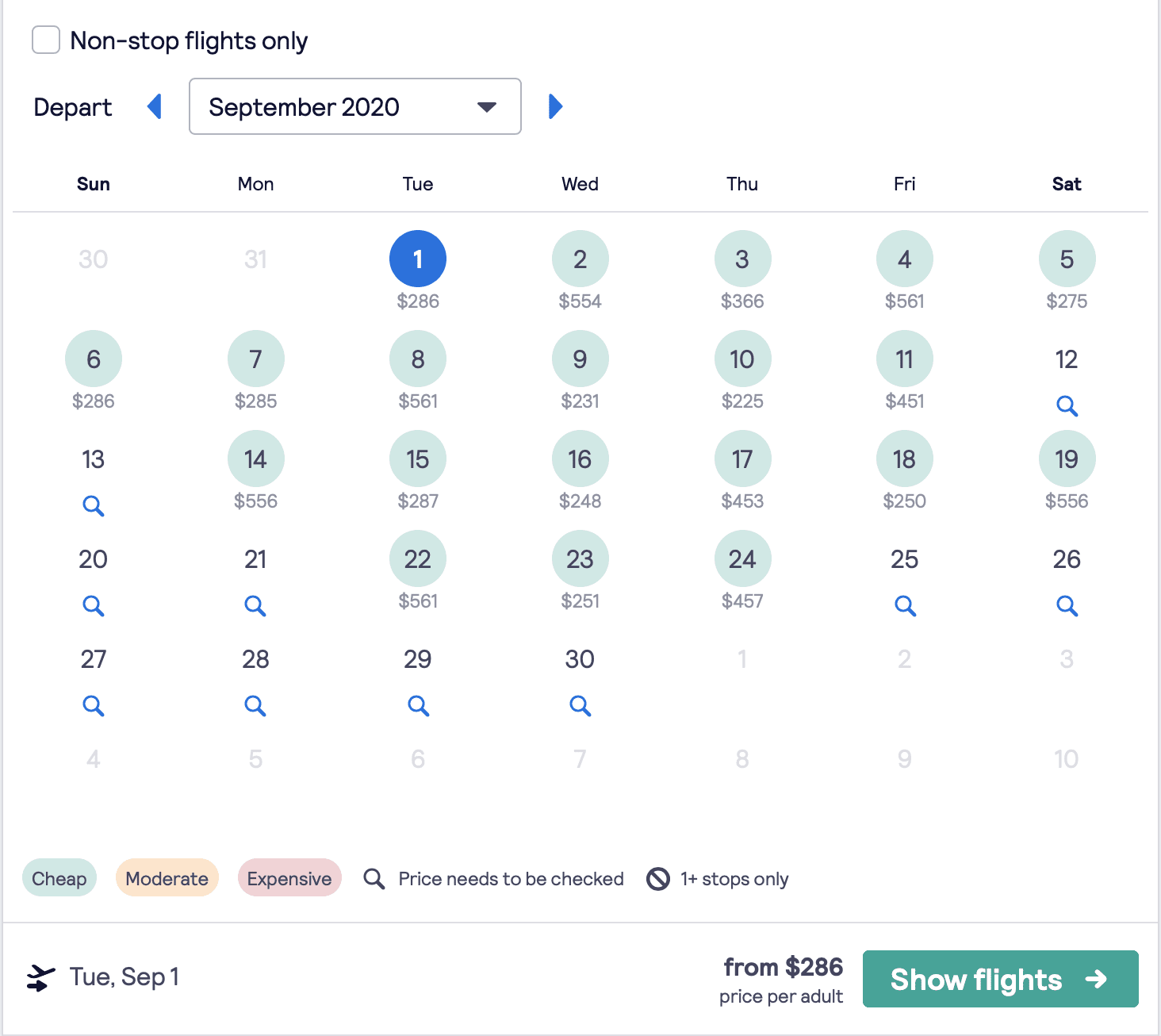The image displays a flight search interface against a white background. At the top, there's a calendar with a checkbox labeled 'Non-stop flights only.' Below this, to the left, is a 'Depart' label accompanied by a left-pointing blue arrow, beside which is a dropdown menu displaying 'September 2020.' A right-pointing blue arrow follows the dropdown.

The calendar layout below shows the first of September starting on a Tuesday and the last day, the 30th, ending on a Wednesday. Each day of the month is represented by a light blue circle with the day's number in the center, and flights prices listed underneath each respective day. Days without circles have a magnifying glass icon instead.

Underneath the calendar, there are color-coded boxes indicating price tiers: a blue box for 'cheap,' a pink box for 'moderate,' and a purple box for 'expensive,' with a magnifying glass icon labeled 'price needs to be checked.'

Specific details include a line noting 'Tuesday, September 1st from $286 price per adult.' Finally, at the bottom, there's a dark blue button with white text reading 'Show flights' accompanied by a right-pointing arrow.